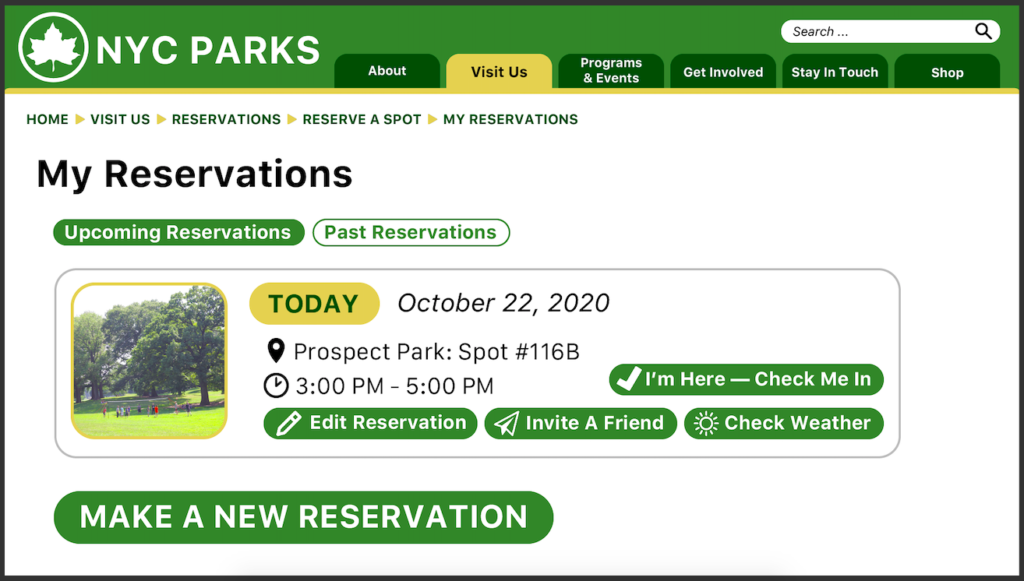The top section features a dark green banner outlined in black, prominently displaying the NYC Parks logo. The logo consists of bold white letters "NYC Parks" adjacent to a white-outlined circle containing a maple leaf. Beneath the logo, the banner includes the following navigation options in white text: About, Programs and Events, Get Involved, Stay in Touch, and Shop. The "Visit Us" button stands out with a gold background and black letters. On the top right corner, there's a search bar labeled "Search" accompanied by a black search icon.

Below this section, the page transitions to a white background featuring navigational links labeled: Home, Visit Us, Reservations, Reserve a Spot, and My Reservations, each written in green with a small yellow arrow pointing to the right, indicating they are clickable. The headline "My Reservations" is displayed prominently in large black letters.

A green banner follows, with "Upcoming Reservations" written in white. Directly beneath, another outlined green banner labeled "Past Reservations" appears in green text.

The main content area features a large gray-outlined rectangle showcasing an image of a grassy field with trees. Overlaying this image, a yellow banner reads “Today, October 22nd, 2020,” followed by details of a reservation: "Prospect Park, Spot Number 116B, 3 p.m. to 5 p.m."

Below the reservation details, four green banners with white text and icons provide additional actions:
1. "I’m Here, Check Me In" with a white check mark.
2. "Edit Reservation" featuring a white pencil icon.
3. "Invite a Friend"
4. "Check Weather" with a sun icon.

The page concludes with a green banner at the bottom that says "Make a New Reservation" in white.